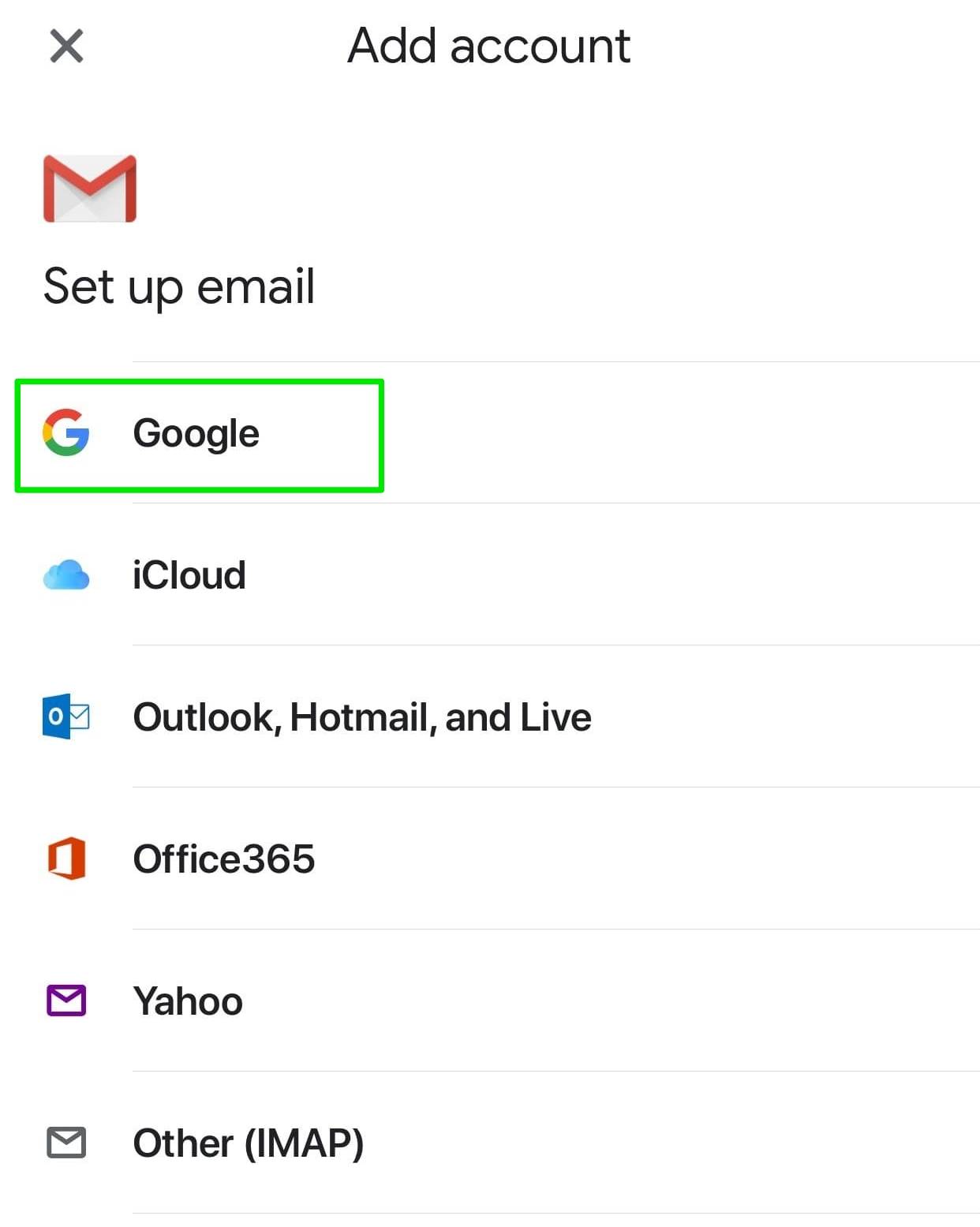A screenshot from a smartphone displays the process of adding an email account within an email application. The interface, set against a white background, is topped with the heading "Add Account" in bold black text. In the top left corner, a small 'X' icon is visible, likely intended to close the setup. Below this, a red and white envelope icon accompanies the text "Set up email." 

A list of various email clients follows, each prefaced by their respective logos. The options, separated by faint horizontal gray lines, include Google (with its multicolored "G" logo), iCloud (marked by a blue cloud icon), Outlook, Hotmail, and Live (denoted by the "O" logo), Office 365, Yahoo, and an "Other" category labeled with "IMAP" in brackets.

Notably, the Google option has been highlighted with an annotated green rectangle, suggesting a recommendation or instruction to select Google.